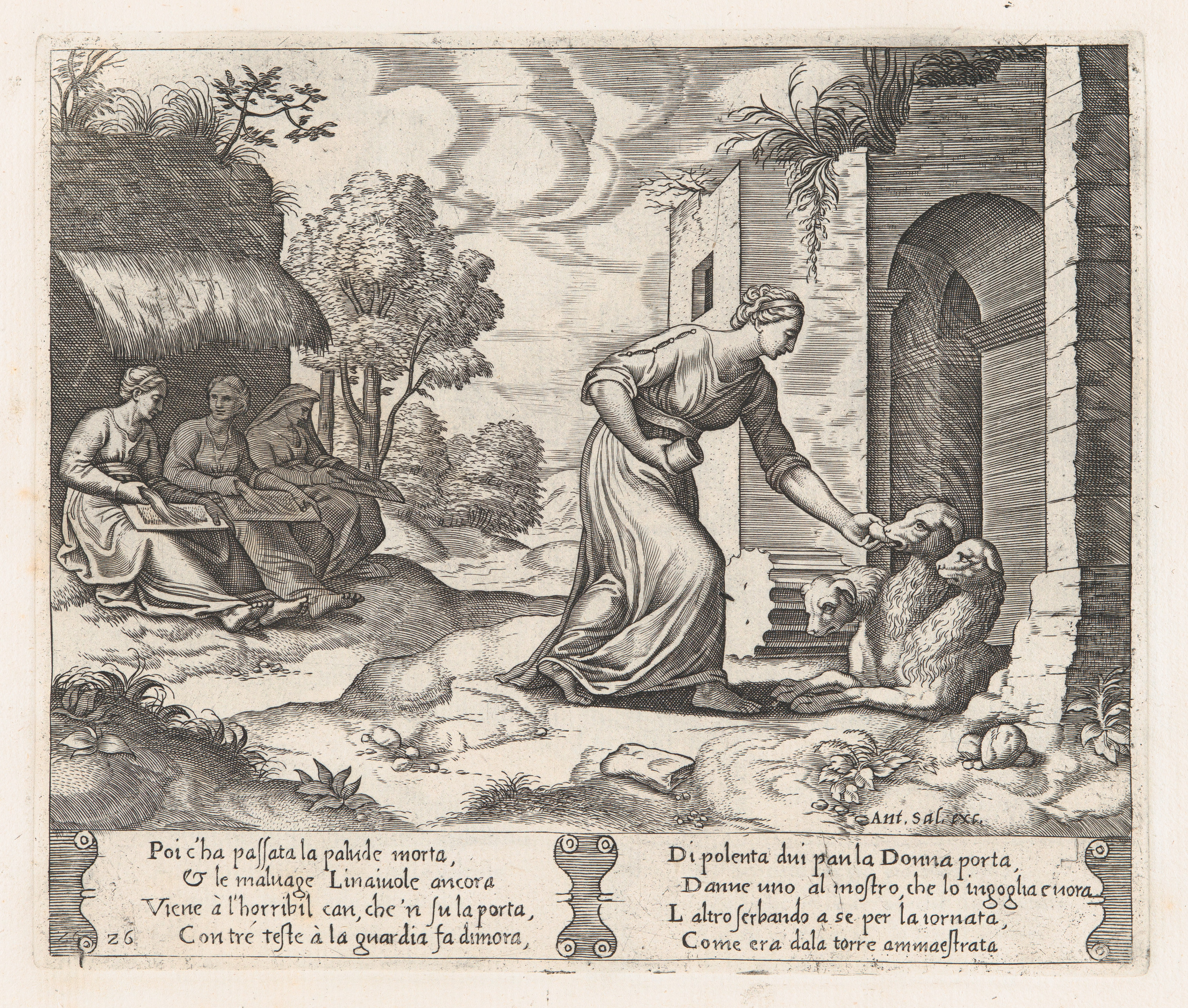This image appears to be a historical reproduction or scan of an old piece of black and white artwork, possibly from the Renaissance era. The central figure is a woman in a robe that covers her body except for her feet, arms, and head. She is depicted bending over and feeding a three-headed creature — likely a dog or sheep — with a loaf of bread in her left hand, while holding a cup in her right hand. Notably, the two heads of the creature that are not being fed appear sad. To the left, three women are seated beneath a shade or hut on a hillslope, engaged in activities like weaving or crafting. In the background, there are clouds in the sky and trees, and on the bottom left of the image, there are visible plants. The detailed text at the bottom of the image, handwritten in what appears to be Italian or possibly Latin, adds to the historical ambiance of the scene, though it is not legible here. The artwork itself is laid on a white background, highlighting its aged, now cream-colored paper which suggests it might have come from an old book.